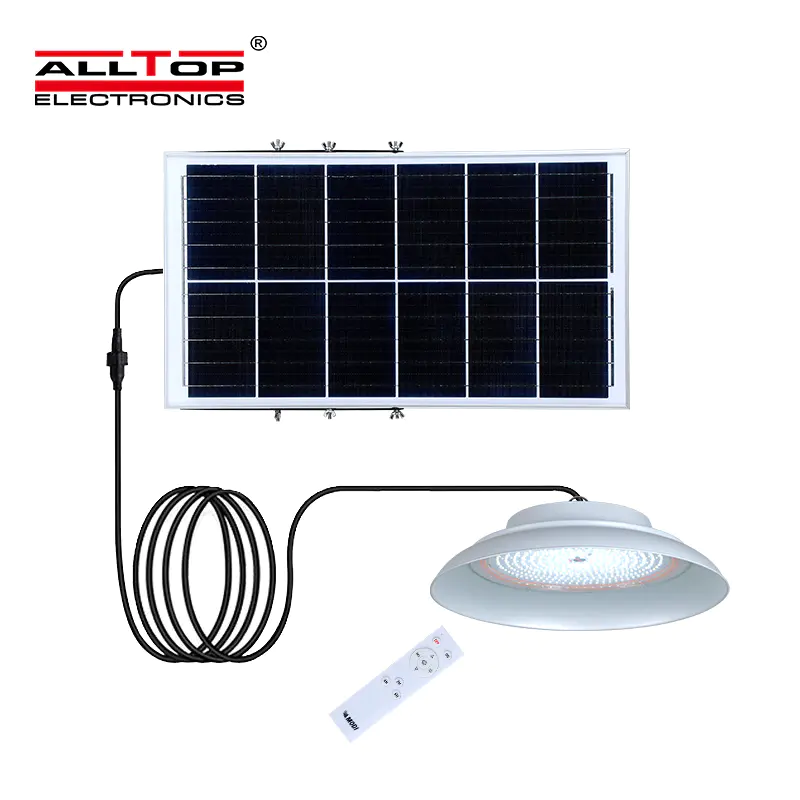The image appears to be an advertisement for a solar-powered light system by All Top Electronics, as indicated by the text in red and black letters in the top left-hand corner. Central to the image is a rectangular black-and-white solar panel encased in a white border, which features several black sections with silver lines running through them. Extending from the left side of the solar panel is a long, coiled black cord that connects to a white, circular light fixture protected by a glass cover. Below the light, in the bottom middle of the image, a white remote control is pointed towards the fixture. The setup suggests that the solar panel powers the light, and the remote is likely used to control the light.